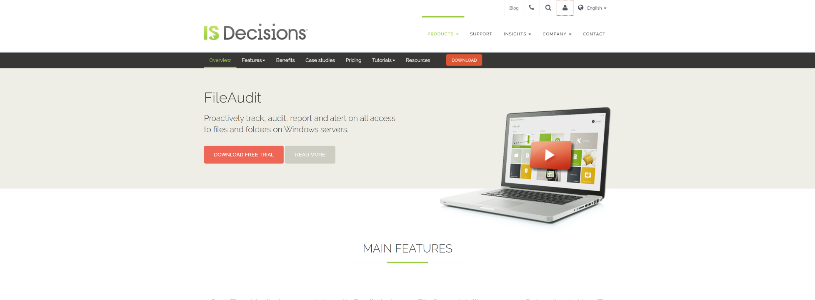Screenshot Description:

This screenshot captures the homepage of a website named "IS Decisions," as indicated by the logo displayed in the top-left corner. Directly beneath the logo, there appears to be a category list, although the text is too small and slightly blurred, making it unreadable. On the left side of the page, there is a section titled "File" with a two-line description below it, which is also too small and indistinct to decipher clearly. To the right of this section, there are two buttons: a peach-colored button and a gray button, though their labels are not legible due to the resolution. Centered on the page is an image of a laptop, prominently displaying what looks like the YouTube logo on its screen.